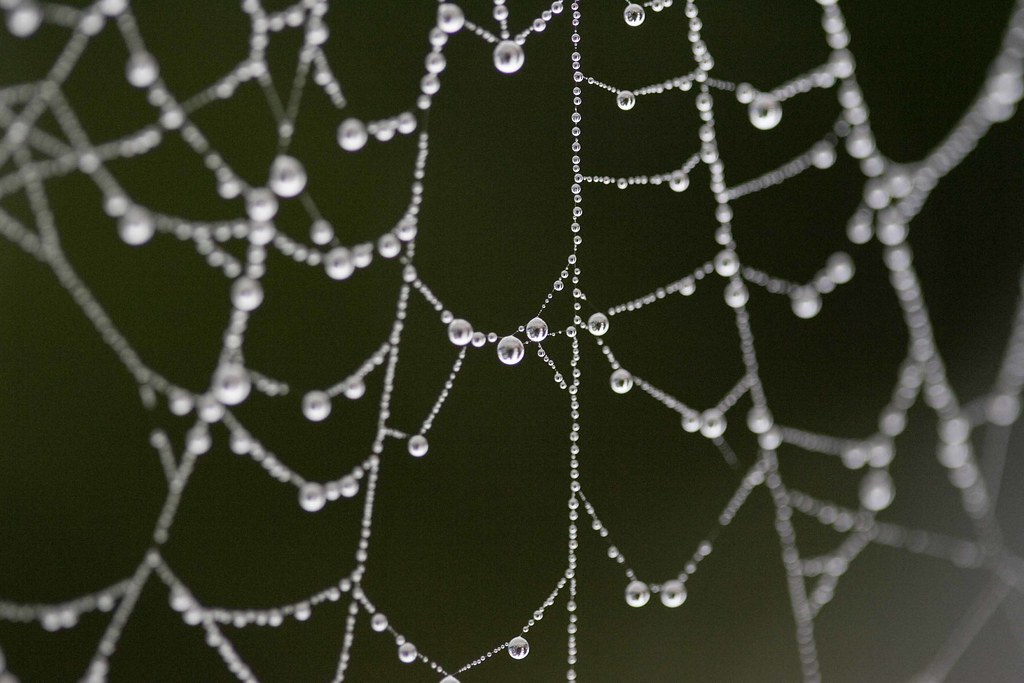This black-and-white, horizontally aligned, rectangular image presents a close-up photograph of a spiderweb adorned with water droplets. The background is a solid black, slightly blurry in the lower right and upper left corners. The spiderweb, primarily in focus at the center, consists of vertical strands made of tiny silver beads or closely linked water droplets. These strands descend vertically down the middle and angle outwards on the left and right sides. The beads on these outer strands appear more gray and blurry compared to the sharp, silver beads in the center. Attached to these vertical threads are larger, transparent gems or water droplets, creating the appearance of a jewel-studded web. The structure is somewhat disordered, with the vertical strands clearly visible, but the horizontal strands less uniformly connected.